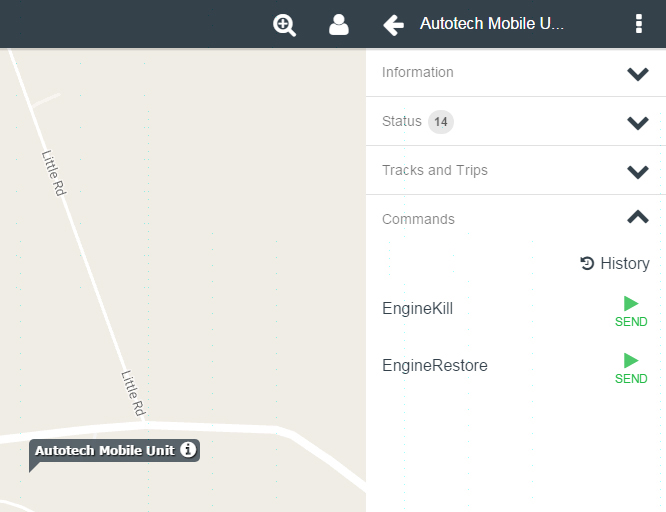Screenshot of the Autotech Mobile Unit Application Interface:

On the left side of the screen, a map is displayed with "Little Road" as the only labeled street. At the bottom left of the map section, an icon representing an Autotech mobile unit is shown, accompanied by a small information icon.

At the top of the interface, a gray bar spans across the screen. From left to right, it contains the following elements: a magnifying lens with a plus sign for zooming in, a user profile icon, a leftward-facing arrow leading to "Autotech Mobile U" followed by an ellipsis, and, on the far right, an icon featuring three dots and a column-like pattern, likely serving as access to additional settings or options.

To the right of the map, several tabs are visible, labeled "Information," "Status," "Tracks and Trips," and "Commands." The "Status" tab indicates 14 notifications or updates, while the "Commands" tab is currently open. Within the "Commands" section, the history is empty, but there are two actionable buttons: "Engine Kill" and "Engine Restore." These options allow the application user to send commands to either disable or re-enable the engine of the Autotech mobile unit.